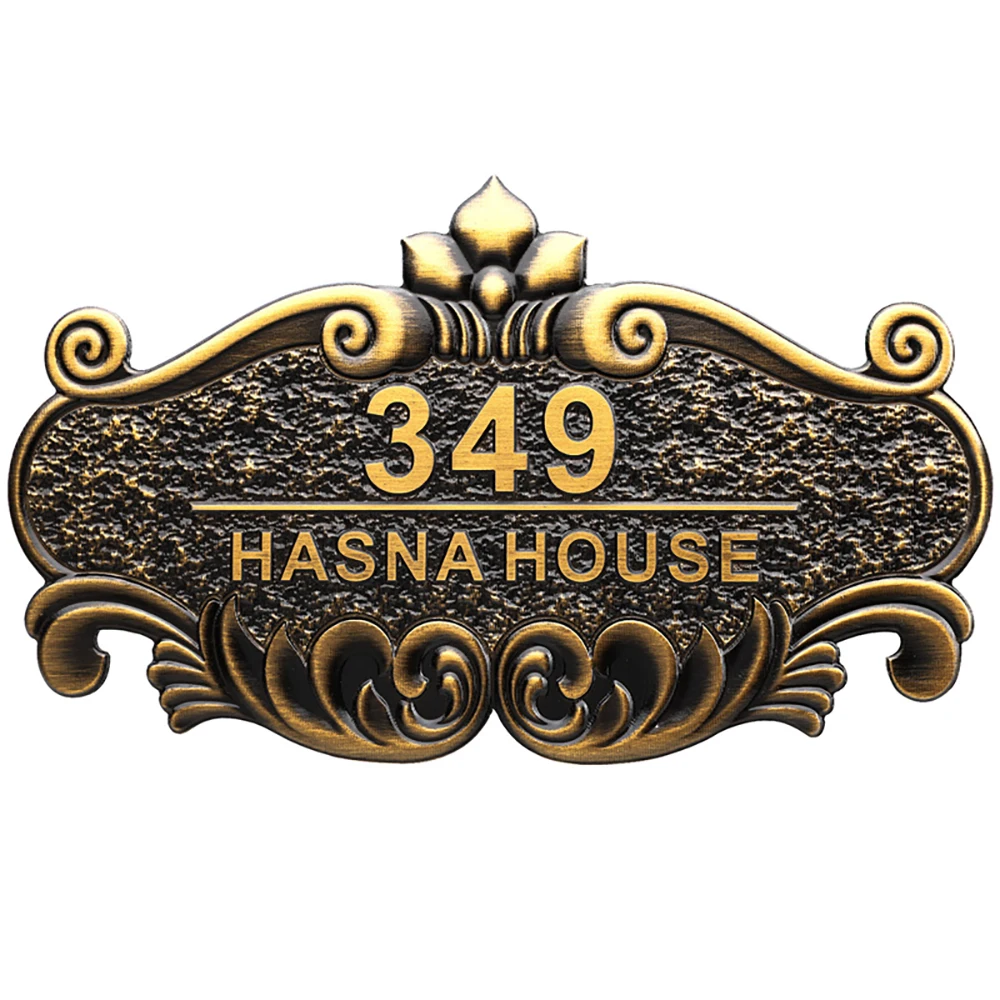This photograph features an ornate brass address plaque reading "349 Hasnah House." The plaque is meticulously crafted, with a golden color accentuated by a black patina that highlights its textured and rough interior surface. The numbers "349" and the letters of "Hasnah House" are smooth, clean, and gleaming, standing in clear contrast to the background texture. The plaque has an oval shape with rounded edges and is adorned with intricate metalwork. At the top, a half-flower embellishment is flanked by wave-like and curly lines reminiscent of a mustache. Additional decorative flourishes, including leafy and wave patterns, extend from the bottom. The plaque appears to be designed for outdoor display, likely affixed to a building to indicate its address. The image shows the plaque against a white background, possibly digitally edited to remove any shadows.